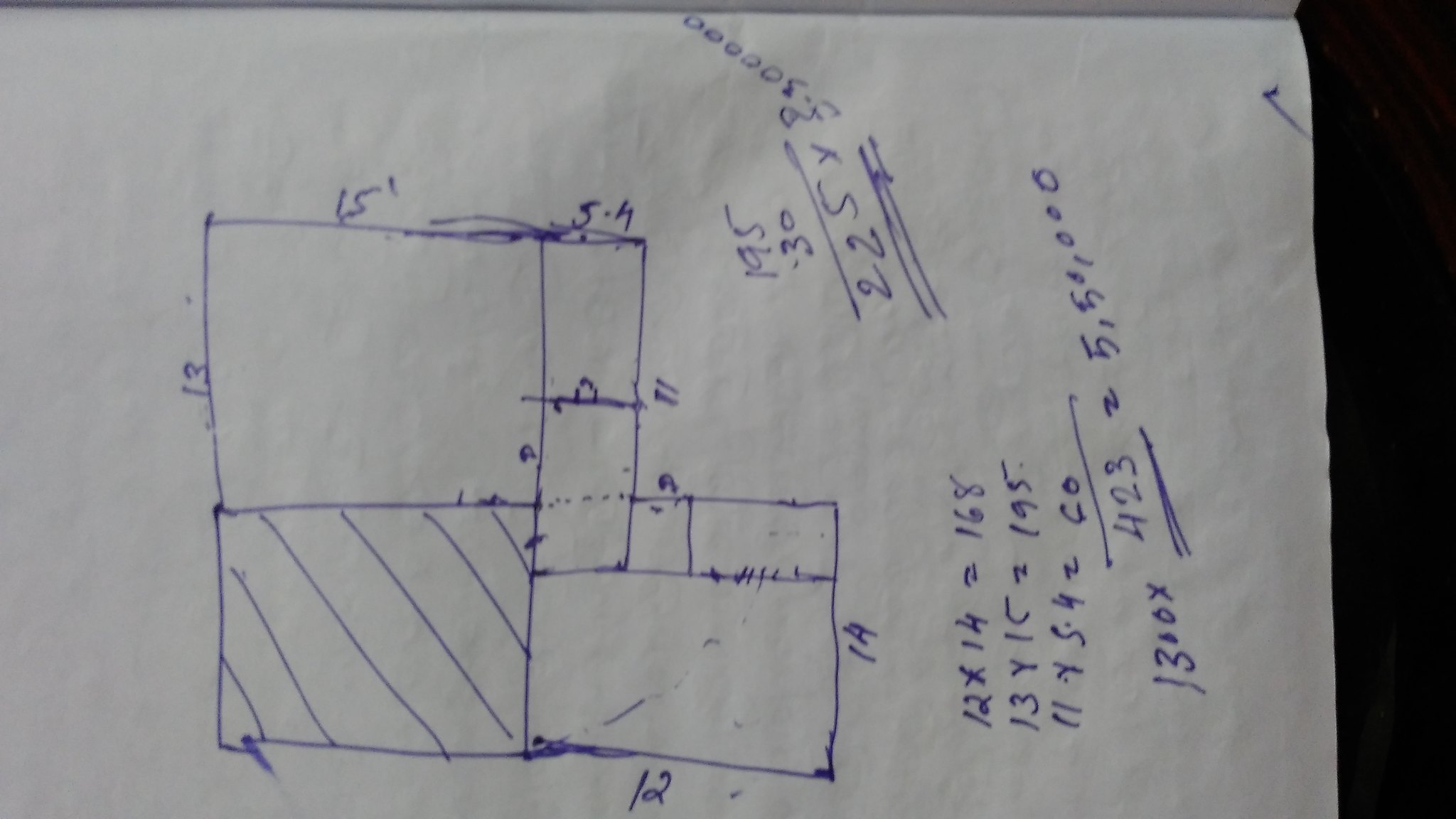This image showcases a detailed hand-drawn architectural sketch, likely depicting the floor plan of a building under development. The sketch includes precise dimensions and notations for various sections, featuring an L-shaped layout. One segment of the drawing specifies dimensions of 15 feet by 13 feet by 11 feet by 12 feet, indicating the measurements of a particular room or area. Additionally, there are numerical annotations such as "12 by 14 equals 168 feet," "13YC equals 195," and "11YS4 equals 60 feet," though some values and calculations, like "1300 by 423 equals 5,500 feet," are somewhat unclear. The upper portion highlights another room labeled as 13 feet by 15 feet, while another part mentions 12 feet by 14 feet, creating a somewhat ambiguous understanding of the areas. The sketch features slanted horizontal lines, adding texture and depth to the drawing, though the exact purpose of these lines is not entirely clear. Overall, the image captures the meticulous planning and calculation involved in the architectural design, albeit with some ambiguities in certain measurements and annotations.